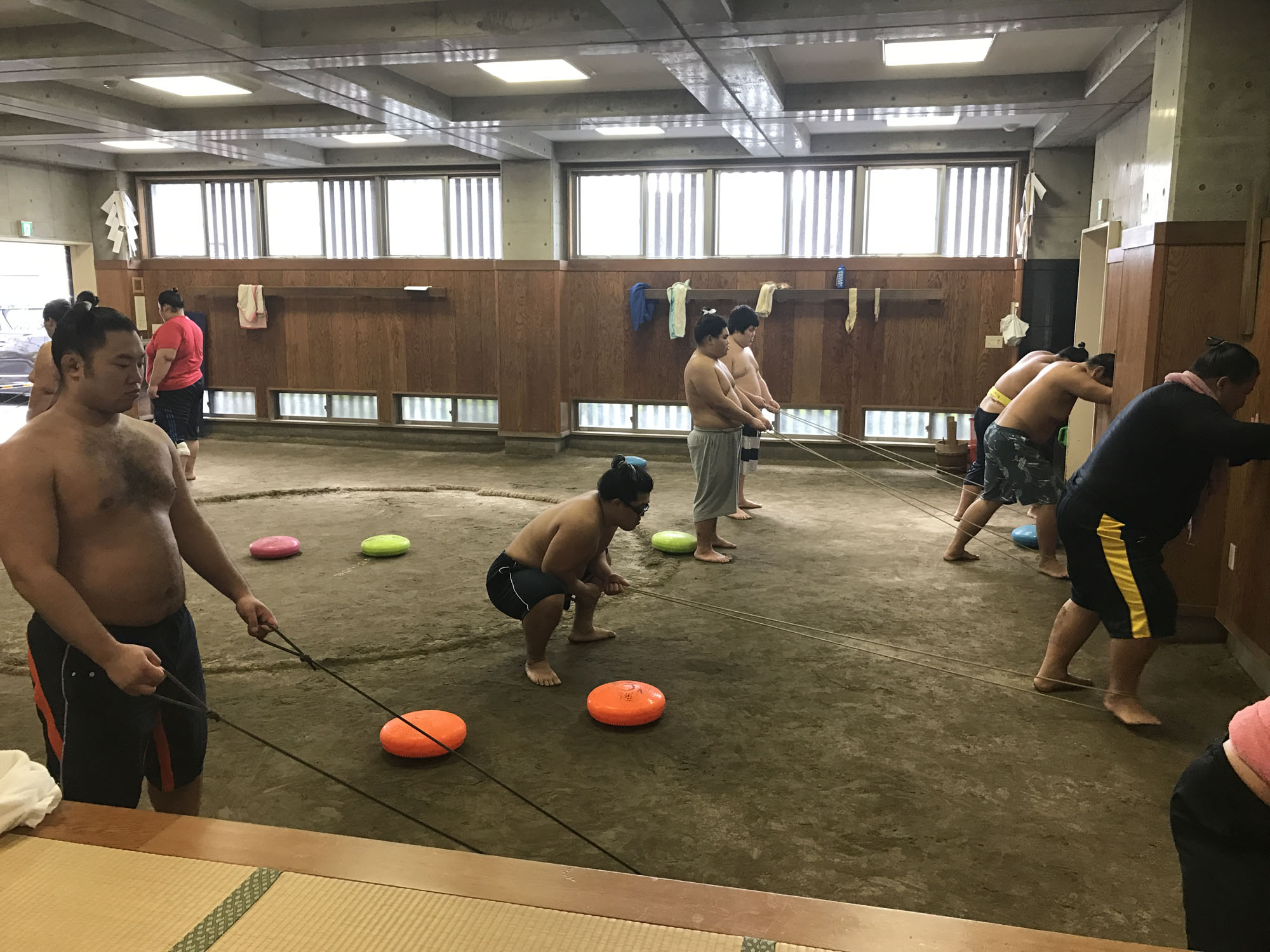The image depicts an interior scene of an Asian training facility, likely a dojo, with a dirt floor and a large circular ring in the center for practice. The setting has a wooden background with windows and a relatively low ceiling. The room is occupied by several shirtless men of Asian descent, appearing to be sumo wrestlers, engaged in a training exercise. In the foreground, there are pairs of men where one individual has ropes tied around his ankles and is leaning against a wall, seemingly pushing against it, while another man stands around ten feet behind him, holding the other ends of the ropes to provide resistance. This exercise appears to be intended to strengthen leg muscles. Scattered across the floor, both inside and outside the ring, are various round, plastic-covered weights in different colors, including orange, blue, green, red, and purple, resembling oversized Mentos.